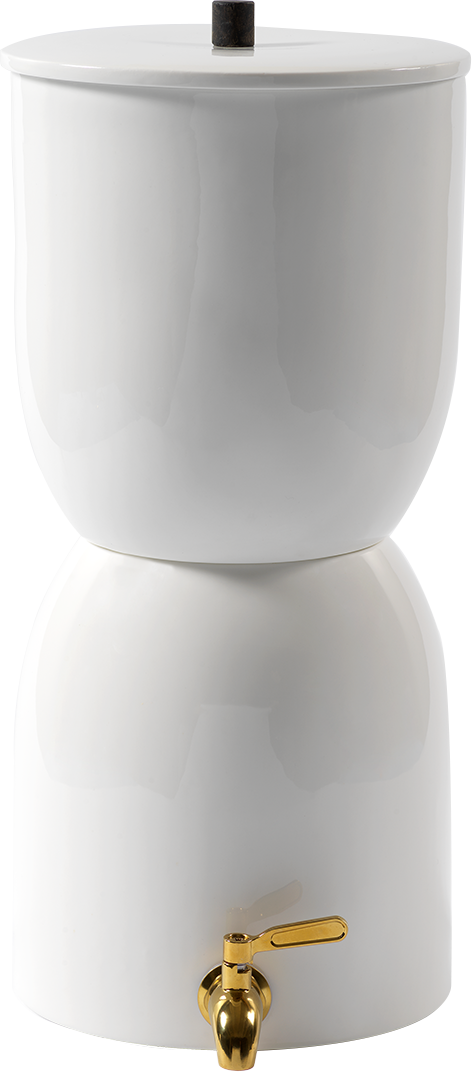The image depicts a two-tiered, shiny white ceramic water purifier or dispenser. The design features a top and bottom section that mirror each other, with the top part resembling the lid of a toilet tank, complete with a flat circle top and a small black knob in the center. Both sections have a cylindrical shape that tapers inward towards the middle before flaring out again. The bottom section has a glossy, ivory-white appearance and ends with a flat circular base. A golden spigot, equipped with a lever for dispensing water, is situated right in front at the bottom center. The lever faces to the right but is designed to be turned forward to release the contents. The glossy finish and smooth contours of the dispenser give it a polished, elegant look.